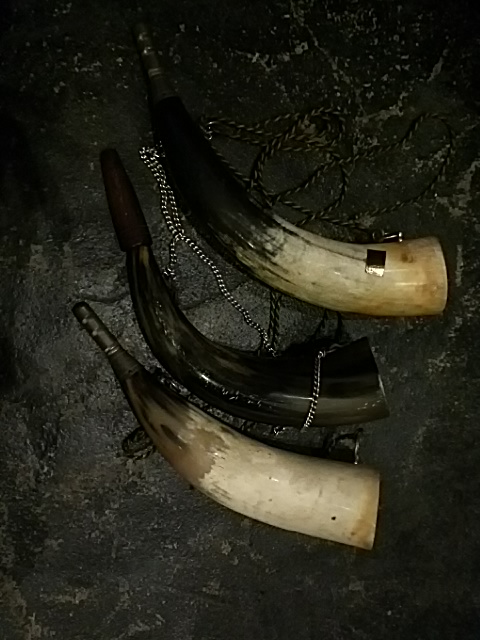The image portrays three ornate horn-shaped tusks, each featuring intricate mouthpieces and silver chains for carrying. The central horn is entirely black, while the two outer horns are ivory or bone-colored with darker detailing closer to the mouthpieces. All three objects rest on a black, patterned surface, possibly suggesting a museum display. The juxtaposition of the cream and black horns against the dark background makes them stand out vividly. These historical-looking artifacts are reminiscent of those seen in old-time period pieces like "Vikings," and they appear to be ceremonial horns used for announcements, rather than personal items.